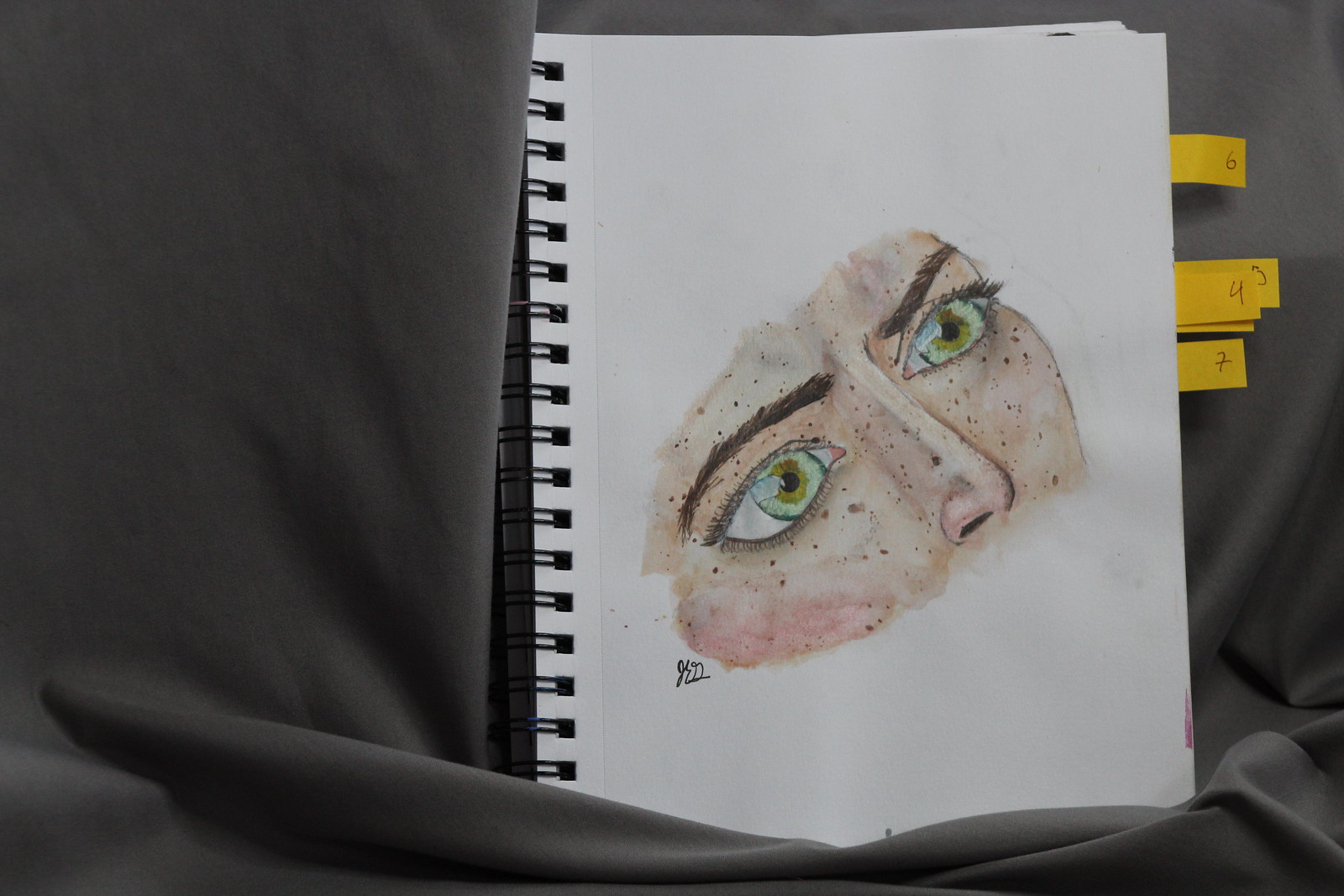In this horizontally-oriented photograph, an artist's sketchbook is prominently displayed standing upright and leaning against folded black fabric. The black fabric partially encircles the bottom of the sketchbook, adding texture and contrast.

The sketchbook, opened to reveal a drawing, features a black spiral binding along its left side. The artwork within the sketchbook depicts a close-up of a human head from the forehead to just below the nose, reminiscent of a mask covering only the eyes and nose.

The face in the artwork is flesh-toned with light green eyes, suggesting a Caucasian individual. The gender is ambiguous, and the face is turned upward, providing a diagonal view from the lower left to the upper right. The artwork's details are meticulously rendered, showcasing brown freckles scattered across the face, large almond-shaped eyes with dark brown, thin eyebrows, and a straight nose with deeply shaded nostrils. Each eyelash is carefully drawn, highlighting the beauty of the eyes with their black pupils, light green irises, and a light blue ring around the edges.

In the lower left corner of the sketch, the artist's initials "RG" are neatly inscribed in cursive.